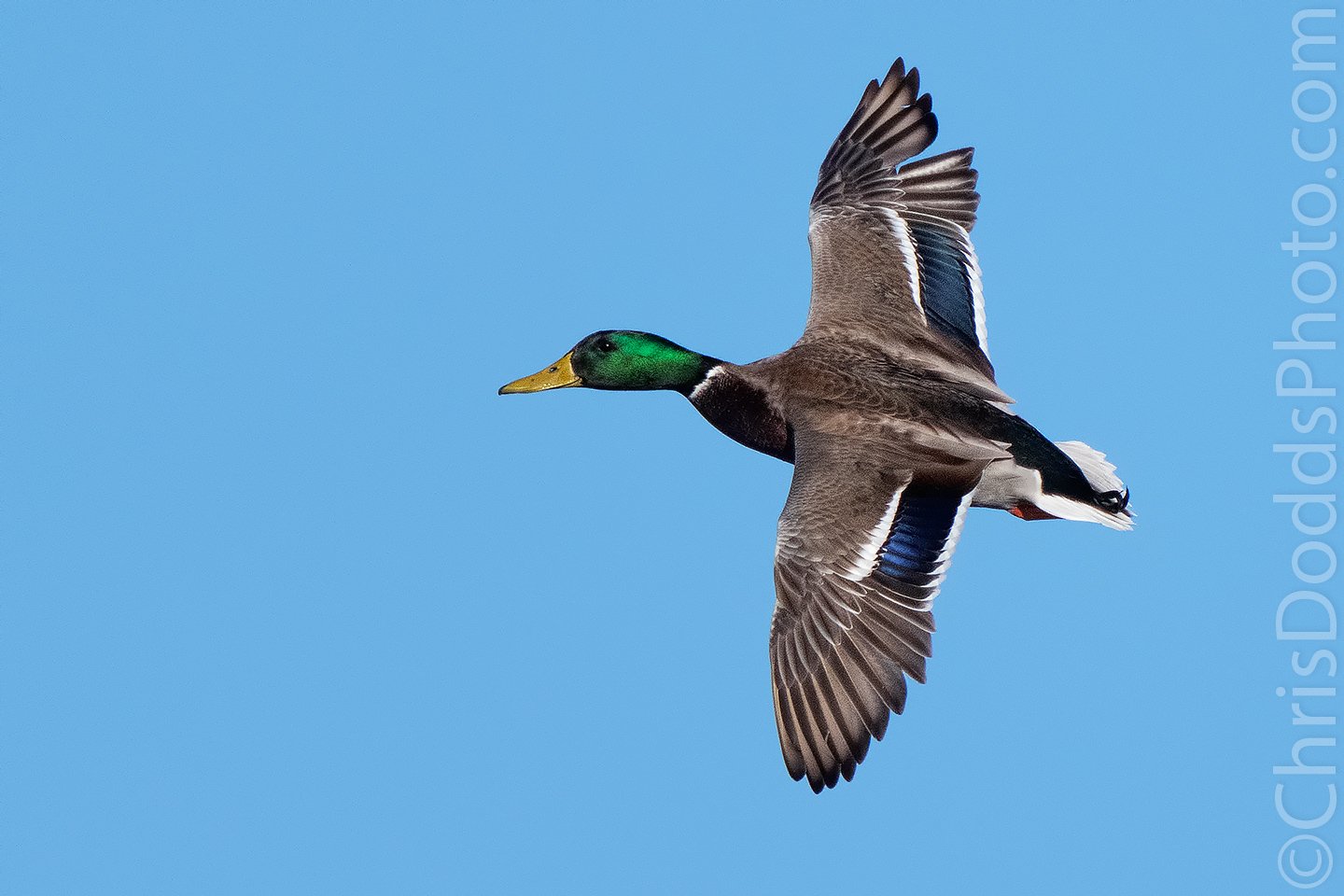A mallard duck is elegantly soaring through a completely clear, blue sky. The bird's wide wings are detailed with a prominent pattern: grayish on the top, transitioning to blue with thin white stripes on the underside. The mallard's distinctive head is a vivid green, complemented by a bright yellow beak. A white ring encircles its neck, leading to a predominantly brown body with notable gray and blue feather accents. The tail feathers are arranged with blue in the center and white on the outer edges. This horizontal, rectangular photo prominently features the text "chrisdonaldphoto.com" on the right side, vertically.